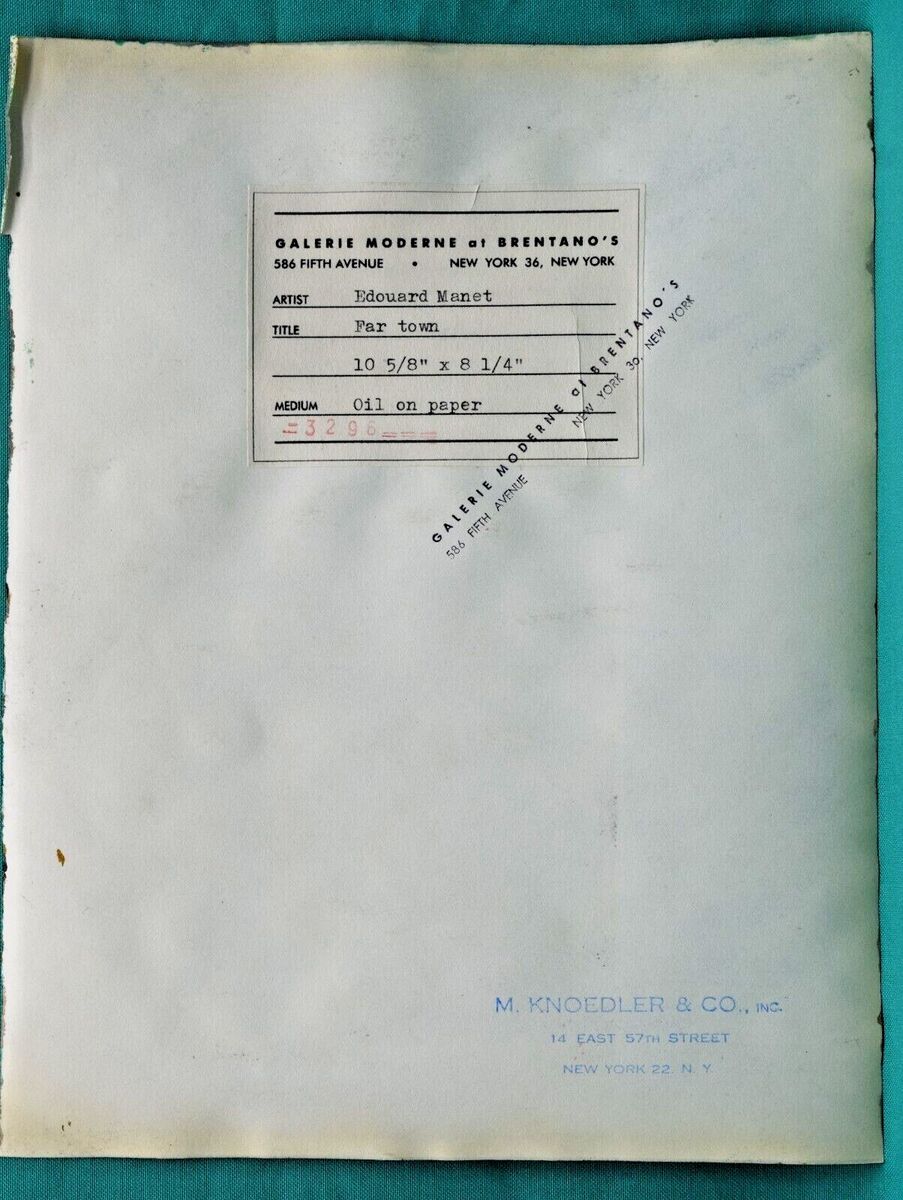The image depicts a worn, slightly stained piece of paper sitting atop a blue-teal tablecloth. The paper appears to have been torn from a book or document and features several key elements. A prominent label with a white background and a black-outlined rectangle at the top indicates the gallery name: "Gallery Modern at Brentano's, 586 5th Avenue, New York." The label also details the artist Edouard Manet, misidentified as "Edward Manet" or "Edward Monet" in some accounts, and specifies the title "Fartown," with dimensions listed as 10 5/8 inches by 8 1/4 inches, and the medium as oil on paper. The paper bears a red stamp reading "3296," and another stamp in blue at the bottom right that reads "M. Knoedler and Company, Incorporated, 14 East 57th Street, New York, NY." The overall appearance gives the impression of an older document, adding to its historical intrigue.